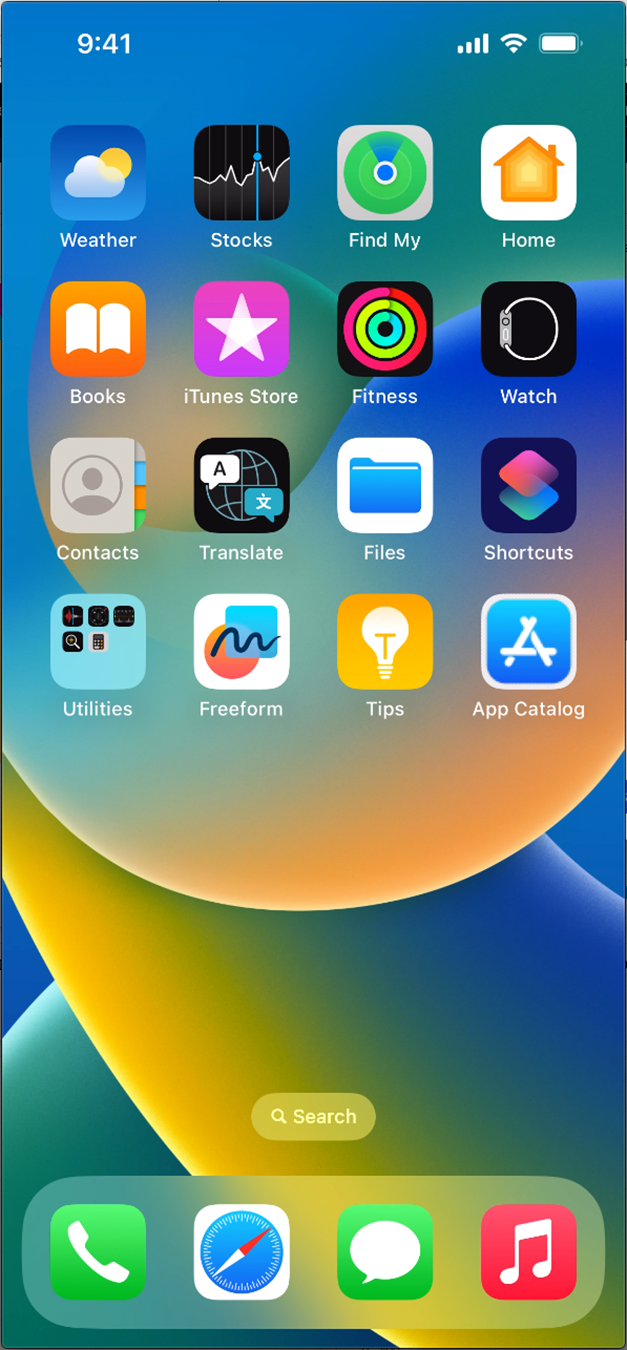A detailed and descriptive caption for the provided screenshot of a smartphone home page:

"A screenshot displaying a smartphone home screen with a layout of app icons. In the upper left corner of the screen, the time is shown as '9:41' in white text. The upper right corner features icons indicating full signal strength, connected Wi-Fi, and a fully charged battery, all in white. The main section of the home screen contains four rows of four icons each. 

The top row's first icon is a blue weather app displaying a cloud with the sun behind it. Following that is the Stocks app with a black icon featuring a yellow zigzag line. Next is the 'Find My' app, represented by a green circle with a blue dot in the center. Adjacent to this is the Home app, marked by an orange icon with a house silhouette.

In the second row, the first icon is for Books, shown by an orange icon with white open pages. Next to it is the iTunes Store, indicated by a pink icon with a white star. The following Fitness app icon is black with concentric circles in red, green, and yellow. Lastly in this row is the Watch app icon, which is black with a white circle.

The screen includes another set of icons, each color-coded and vividly depicted. 

At the bottom of the screen, there is a horizontal strip of four additional key icons: 
- A green phone app icon with a white phone outline is in the bottom left corner.
- Next to it is the Safari browser, symbolized by a blue circle with a compass, with red and white arrows pointing in different directions.
- To the right is the Messages app, shown as a green icon with a white speech bubble.
- Finally, the Music app is marked by a red icon with a white musical note in the center."